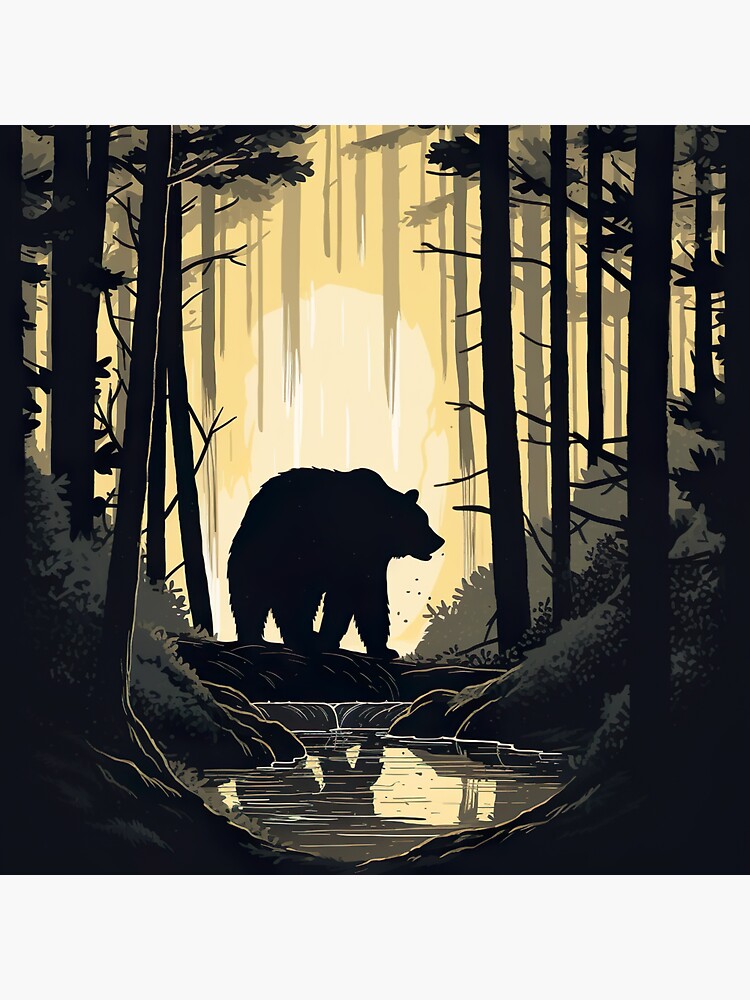The digitally created square image, framed by a white border on the top and bottom, portrays an outdoor forest scene with a profound use of shadows and light. Dominating the center of the image is a silhouetted black bear in a profile stance, making it the focal point of the artwork. The backdrop showcases an orange sun set against an orange-gradient sky that transitions from a tan-yellow glow to a bright, light orange, illuminating the bear and casting a striking contrast against it. Faded tree trunks in varying shades of gray loom in the background, their outlines softened by the sunlight. The lower portion of the artwork features a small pond that mirrors both the bear and the vivid sky, adding depth and harmony to the scene. Flanking the pond are dark banks that stretch to the lower corners and sides, adorned with numerous tree trunks and sparse foliage. The overall ambiance is shadowy and moody, accentuated by the interplay of orange light and dark elements.